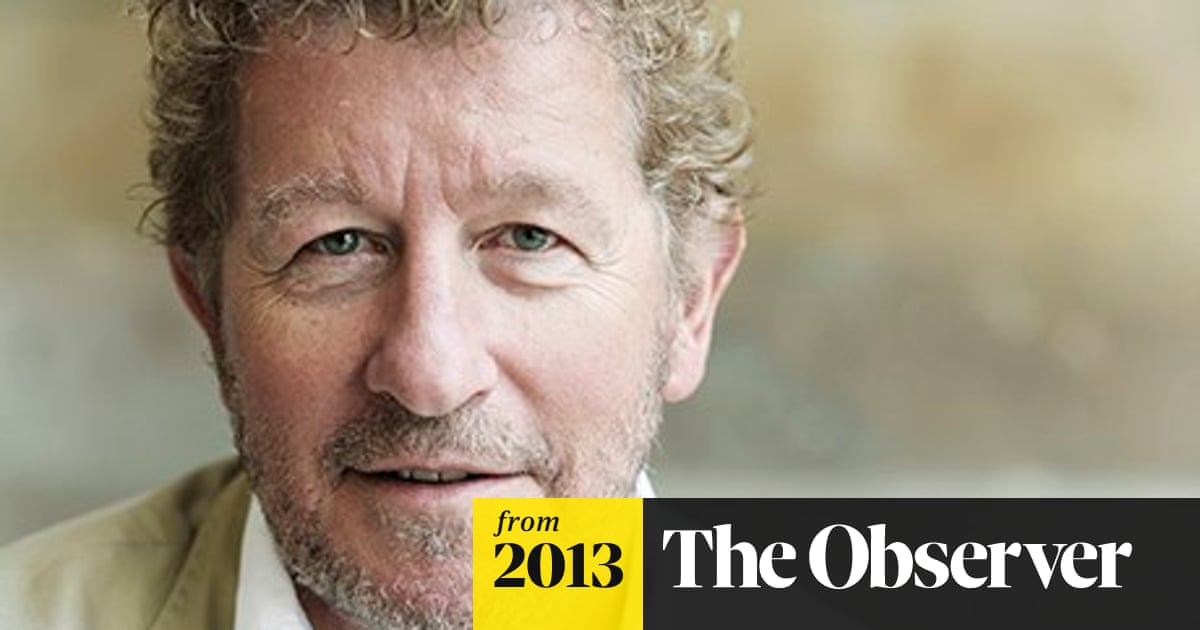The image is an advertisement from The Observer magazine in 2013. It features a close-up of a middle-aged Caucasian man smiling at the camera. He has soft, curly hair that is a mix of brown and blonde, indicating some use of hair product as the curls are not light and fluffy. He sports a scruffy, short beard and mustache with gray and brown undertones. His eyebrows are long and of a similar color to his hair. The man has striking green-blue eyes. He is wearing a tannish-brown jacket over a white collared shirt. The background is blurred, suggesting an outdoor setting with plant life and trees, which directs focus to the man's face and shoulders. The cover prominently displays "from 2013" on a yellow bar and "The Observer" in white text on a black bar.